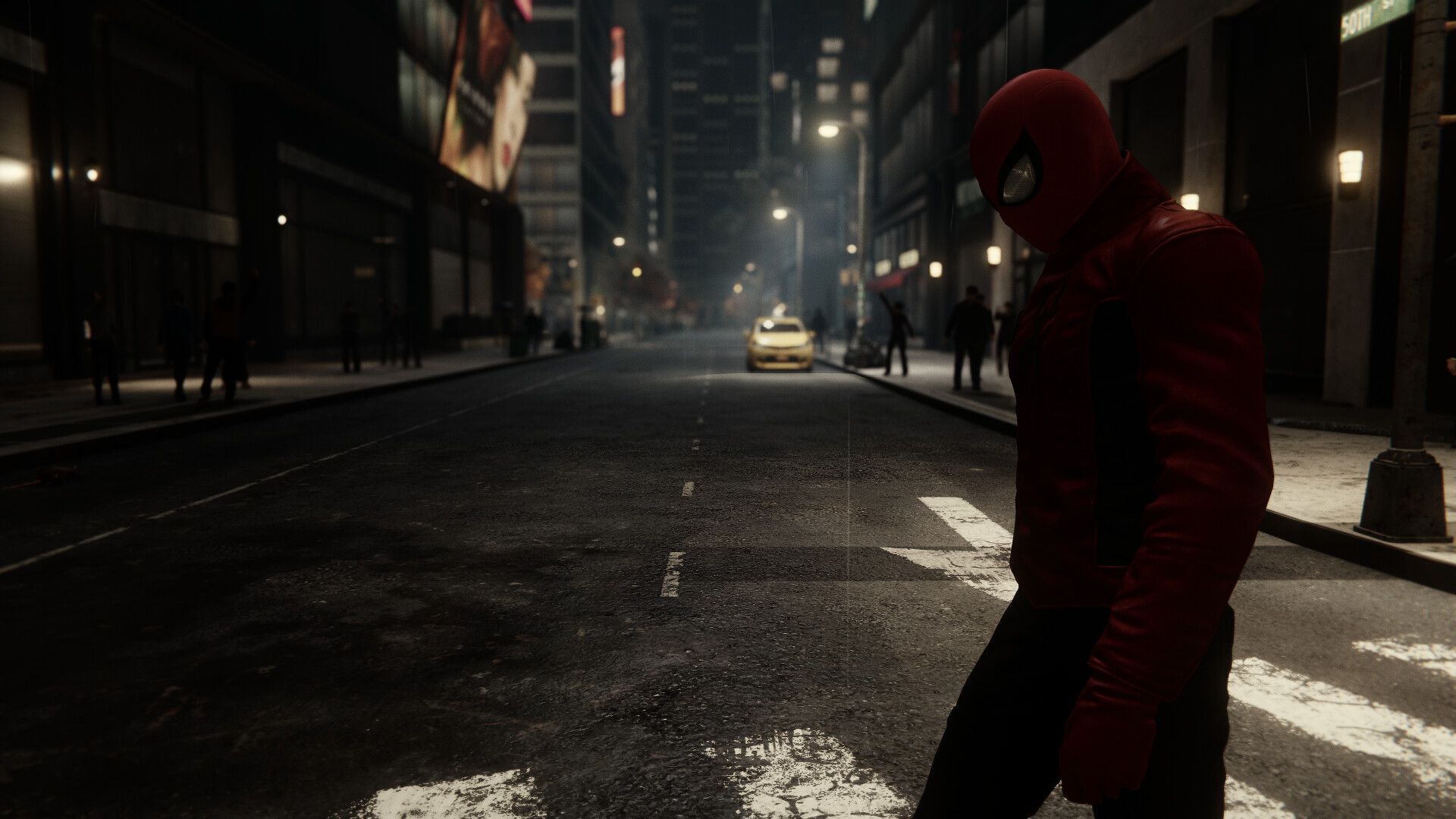In this night-time scene from a video game, Spider-Man is captured walking across a crosswalk. His iconic red head and shoulders, along with his large white eyes, are strikingly visible against the dark surroundings. The rest of his body blends into the night, making only the top portion of his figure discernible. A white taxi is parked on the right-hand side of the street, illuminated by one of several streetlights that line the road. On the left side of the street, an illuminated billboard showcases a woman with pale skin, red lips, and black hair. The background street continues into the distance, with shadowy figures of pedestrians visible on the dimly lit sidewalk.